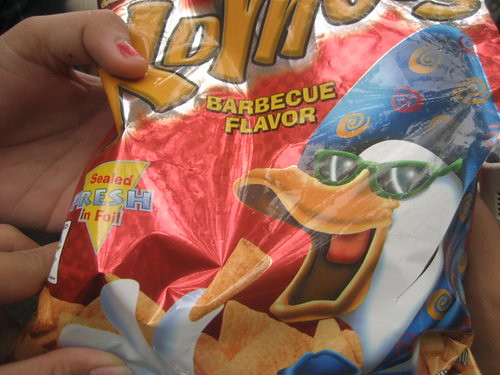The image is a photograph of a crinkled, reflective aluminum-colored potato chip bag predominantly displayed at the center. The brand name on the bag is mostly obscured, with only parts of the letters "K" and "O" visible in yellow bubble letters. The bag features a cartoon white duck with its beak open, appearing to munch on a cone-shaped chip that resembles Bugles. The duck is adorned with green sunglasses and a blue hat or scarf with gold or yellow swirls, giving it a colorful, whimsical appearance. The background of the package is red, and "barbecue flavor" is printed in yellow font below the obscure brand name. To the left of the duck, there is an upside-down yellow triangle with the text "sealed fresh in foil" in red and silver colors. The bag is held by a hand with red fingernail polish, indicating it might be a woman's hand with tanned or brownish skin.